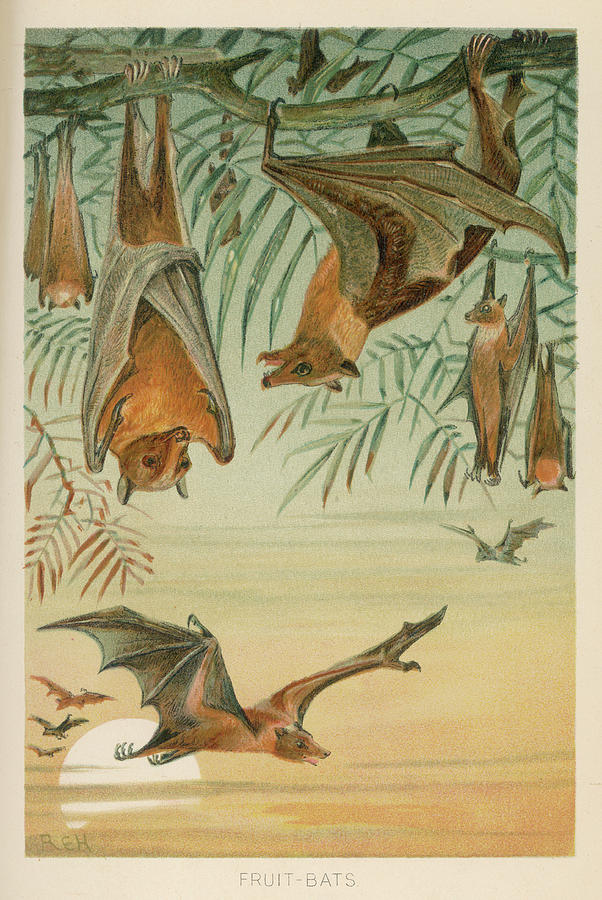The image is a detailed, hand-drawn poster in a botanical style, featuring a variety of fruit bats. In a vertical orientation on an ivory background, the poster shows a composition of bats rendered in oil pastel and watercolor techniques. At the top, a branch with turquoise-green tropical leaves extends into the scene, from which about seven bats hang upside down, their wings wrapped around their bodies and some appearing to engage in conversation. These bats are predominantly brown, black, burnt orange, and gray in coloration.

The sky above transitions from a deep blue at the top to orange as it approaches the horizon, symbolizing either sunrise or sunset, and is dotted with translucent clouds. Below, a bat glides through the air with the sun rising or setting on the bottom left. The overall scene is serene, with an additional bat flying mid-frame and more bats in the background. At the base of the image, the text "fruit bats" is neatly inscribed, along with the signature "R.E.H." This detailed illustration beautifully captures the essence and quiet charm of nocturnal fruit bats in their natural habitat.